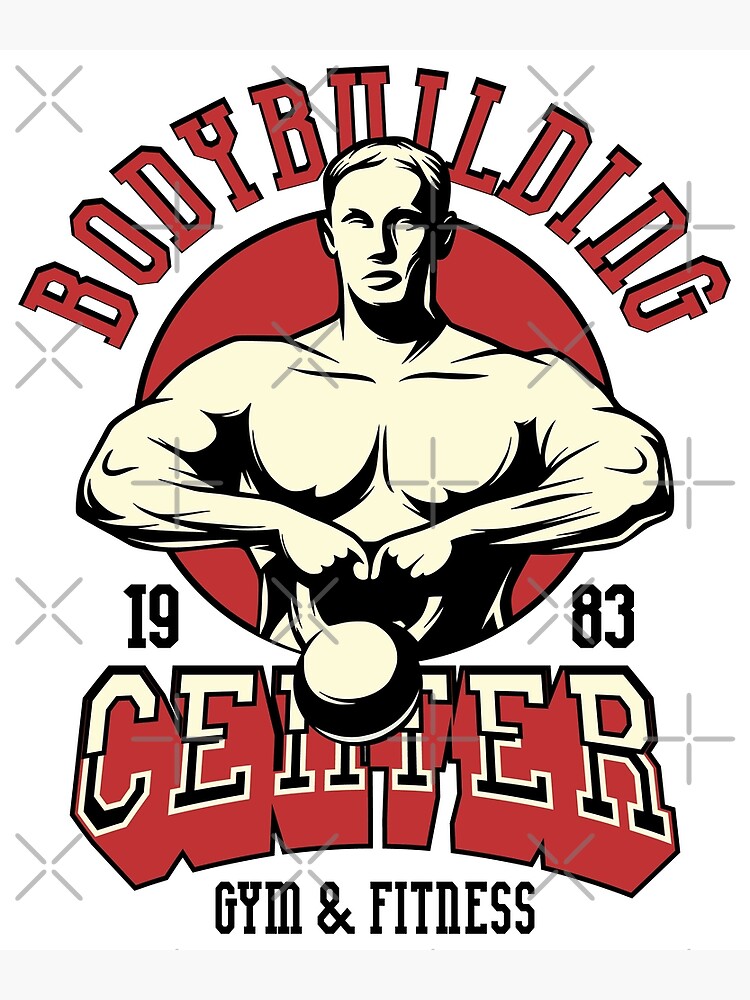The flyer or advertisement features a white background adorned with light gray X's on the left-hand side and light gray plus signs in the middle and on the right, all separated by a small white circle. At the top, in a curved red text, it reads "Bodybuilding," with "Center" written below it. The central image is a detailed drawing of a muscular, shirtless man with short hair, holding a heavy dumbbell in front of him with both hands, his arms positioned up by his chest. Behind him, there is a solid red circle. Below this, the year "1983" is printed in black. At the very bottom of the flyer, the words "Gym and Fitness" are prominently displayed in black.